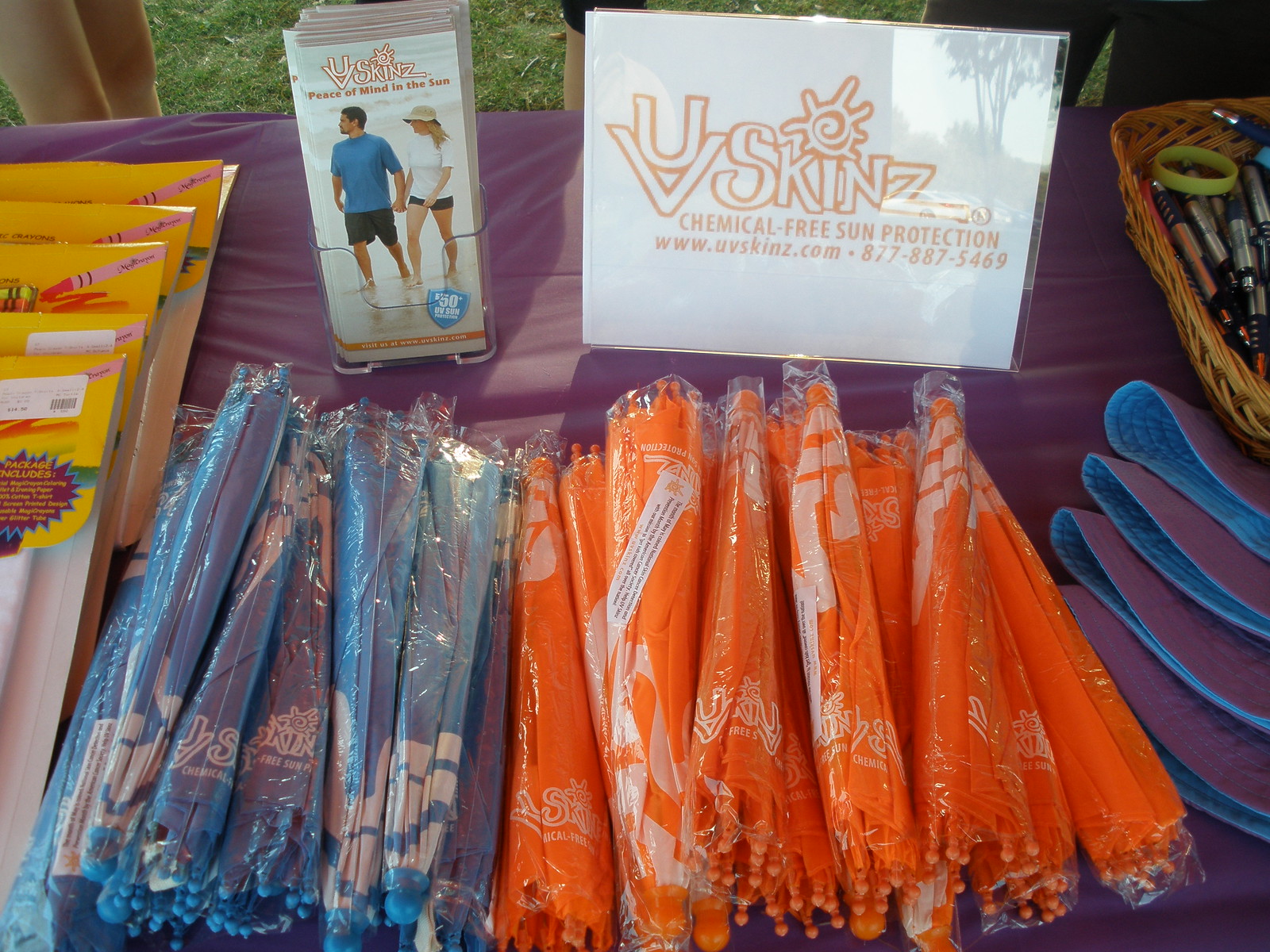This image depicts a promotional display for UV Skins, a brand offering chemical-free sun protection. The display table, adorned with a purple tablecloth, features various items and informational pamphlets. In the upper left corner, a plastic holder contains pamphlets with the titles "Skins," "Peace of Mind," and "The Sun." Beside it, another holder displays a paper that reads, "UV Skins, Chemical-Free Sun Protection," along with the website www.uvskins.com and phone number 877-887-5469. Below this, there are blue and orange items stacked in neat piles, which appear to be wearable umbrella hats designed to protect against sunburn and skin cancer. To the right, there is a stack of purple items and a basket of pins in the upper right corner. The promotional material suggests an alternative to sunscreen, emphasizing the benefits of these wearable sun protection items.